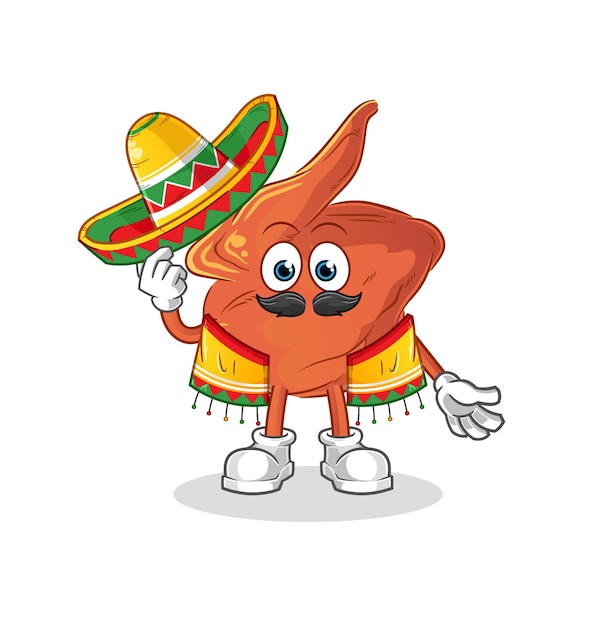The image features a cartoon drawing of a human-like character resembling a chicken wing, colored in a brownish-red-orange hue. This character stands at the center of an otherwise solid white background, creating a stark contrast that emphasizes its presence. The whimsical figure sports expressive blue eyes and a black mustache, adding to its quirky personality. It is adorned with white gloves on both hands, with its right hand holding a colorful sombrero decorated in red, yellow, green, and white with triangular patterns and stripes. The figure also wears matching white shoes and stands atop a round, gray platform. The character's attire includes elements of traditional Mexican clothing, contributing a cultural touch to its distinctive appearance.